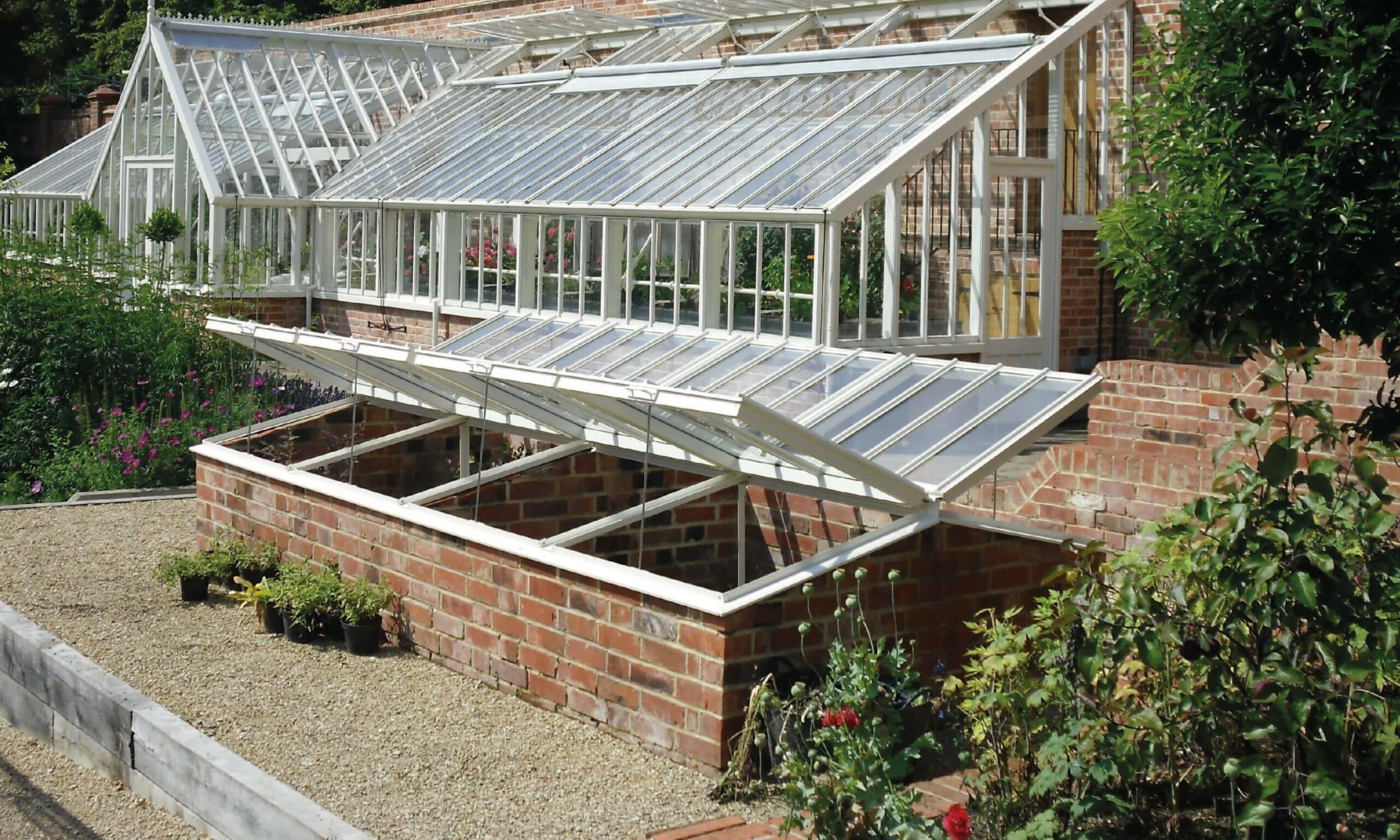This is a bright daytime photograph capturing a greenhouse almost seamlessly attached to a red brick home, creating a cohesive structure. The greenhouse features a white wooden frame with angular lines leading to glass-paneled windows, some of which are propped open. Inside, green plants thrive in the controlled environment. 

Prominently, there is an A-frame section with a double-door entry situated in the middle of the greenhouse. In the foreground, potting beds made of red bricks with glass covers are angled upwards and hovering slightly above the ground. These cold boxes, currently empty, would typically be used for growing plants. 

The ground surrounding the structure is landscaped with tan-colored pebbles and adorned with various foliage, including poppies with visible seed pods on the right and a small garden section on the left. The scene is bathed in bright daylight, enhancing the vivid colors and details of the greenhouse and its surroundings.